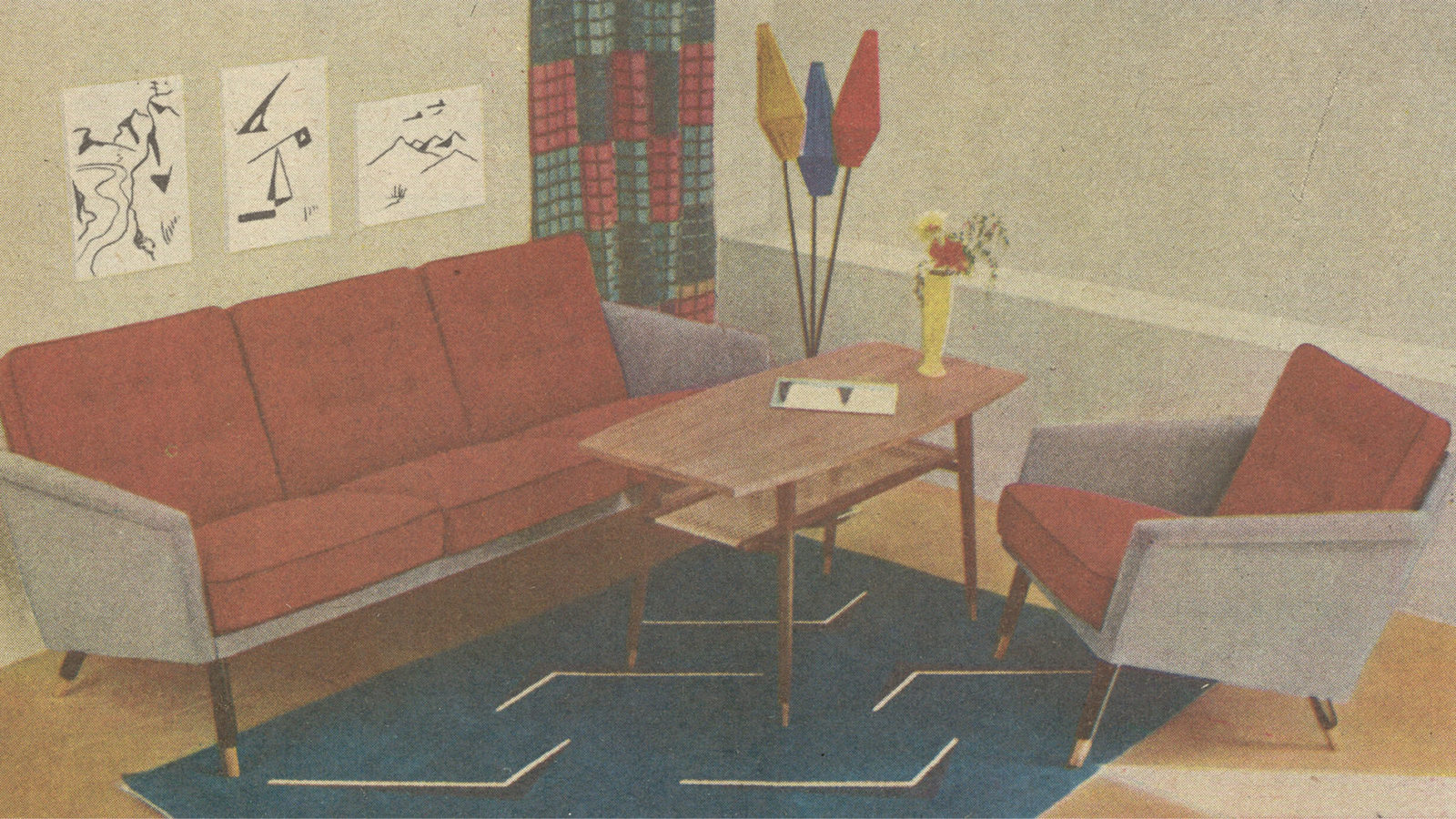This detailed painting portrays a cozy and vibrant living room, possibly a therapist's office, distinguished by its blend of realism and abundant use of color. The room features light grey off-white walls adorned with various drawings made with black markers on white paper, contributing to the room's artistic feel. In the background, a checkered curtain adds more color variability with its red, green, dark green, and yellow squares. 

The floor of the room is brown, partially covered by a blue carpet with white designs. Positioned centrally is a brown wooden table holding assorted items, notably a vase with yellow and red flowers accented by green leaves, and a black-and-white picture. To the left of the table stands a three-seater sofa with grey exteriors and red cushions, complemented by similar single-seater armchairs on the right.

Additionally, the room is illuminated by three lights attached to brown or black stands; the lights at the leftmost, middle, and rightmost positions cast yellow, blue, and red hues, respectively. The interplay of colors like blue, brown, grey, beige, red, and yellow gives this painting a lively yet homely atmosphere, suggesting a typical yet artistic living space, likely an apartment or a therapist’s office.